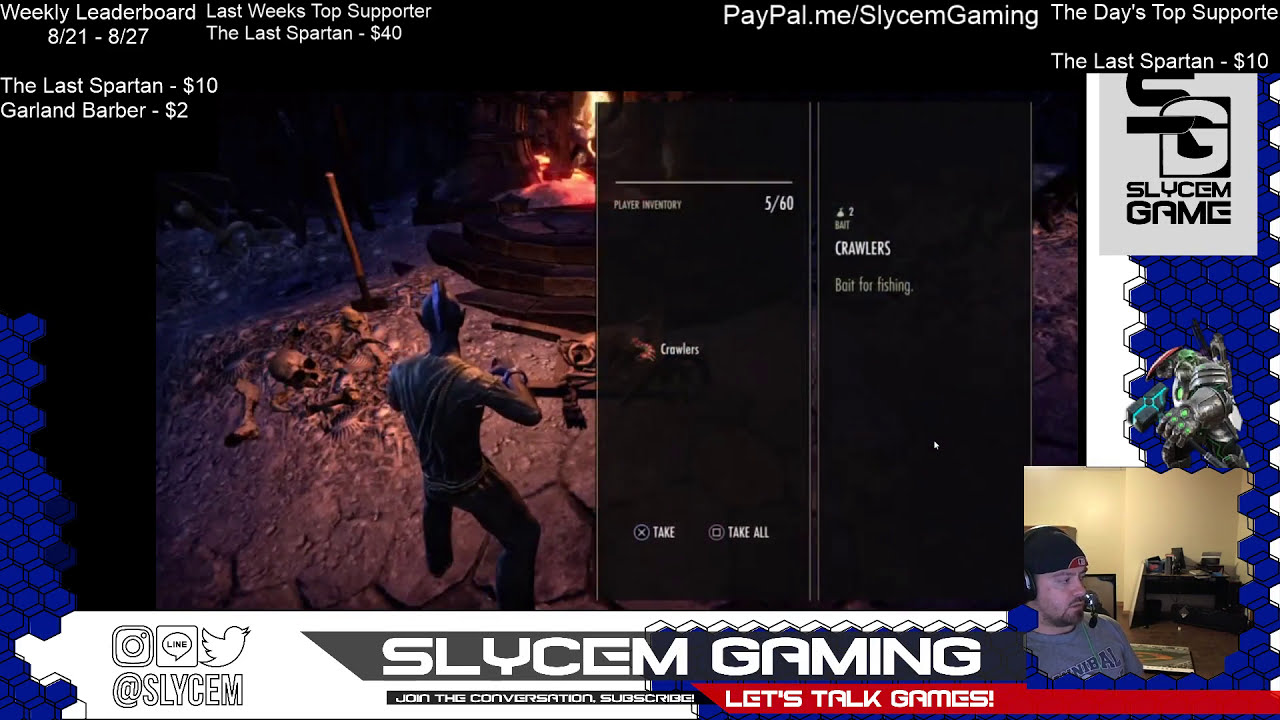The image is a screenshot from a video game stream under SLYCEM Gaming. The central focus is the game itself, which features a humanoid creature with pointed ears and a mohawk, dressed in tattered clothes, standing in a barren, cave-like environment. The character is facing away from the viewer, with a skull, bones, and a shovel on the ground, suggesting an eerie atmosphere. The inventory screen is visible, showing items like "crawlers" and options to "take" or "take all."

In the upper left corner, text reads "Weekly Leaderboard 8/21 to 8/27. Last week's top supporter: TheLastSpartan at $40," followed by current supporter amounts: TheLastSpartan at $10 and Garland Barber at $2. The upper right corner displays "Paypal.me/SLYCEM Gaming" alongside "The day's top supporter: TheLastSpartan $10."

The lower right corner shows a live-view window of the streamer, a Caucasian man with a brown beard, wearing a backward black cap, over-the-ear headphones, and a gray t-shirt. Behind him are shelves with various items. The bottom of the image has a banner with "SLYCEM Gaming" in a white section, encouraging viewers to “Join the conversation. Subscribe,” and a red section stating “Let’s Talk Games.” The entire scene is set against a backdrop featuring blue hexagon patterns, adding a visually complex layer to the presentation.